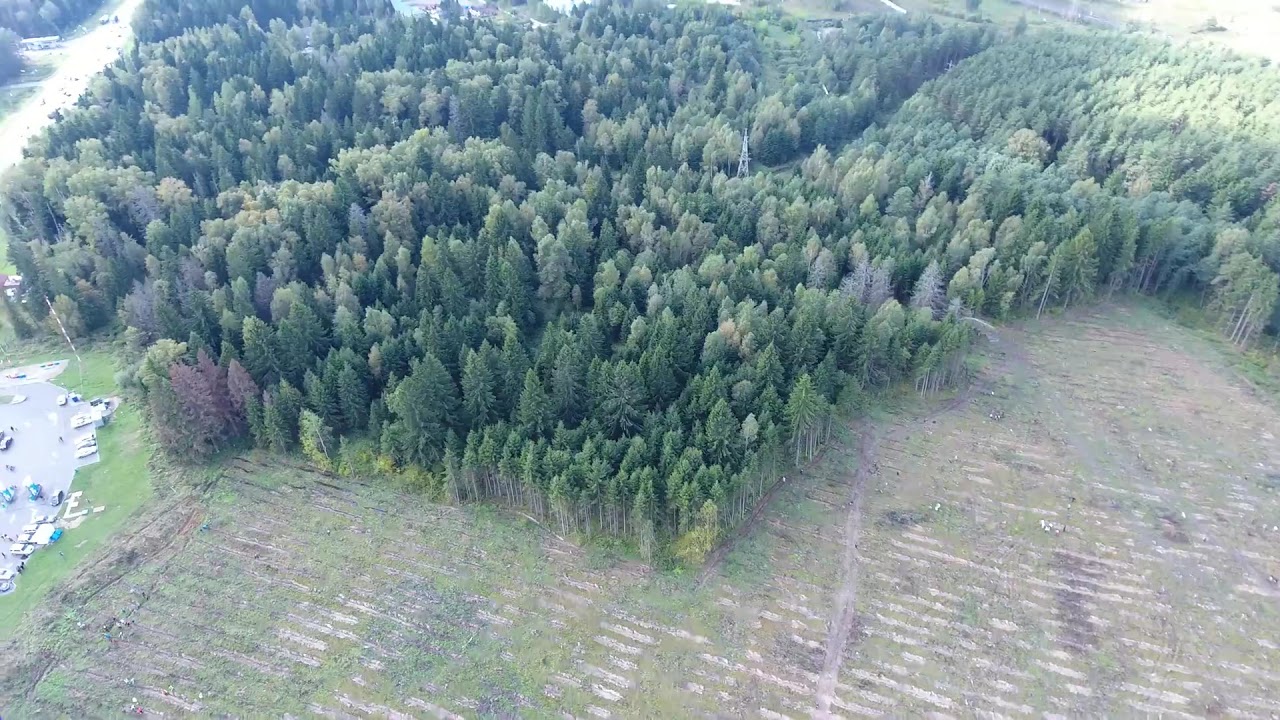The image captures an expansive aerial view of a lush forest environment. The dense canopy of vibrant green trees dominates the top two-thirds of the photograph, with the tree line extending into the center in a tapered fashion. Varied shades of green, interspersed with patches of lighter and purplish-gray foliage, add texture to the scene. Near the edges of the forest, distant tree trunks and barks in light grayish-brown are faintly visible. 

In the lower third of the image, there is an open field with a mix of grass and dirt, exhibiting intricate patterns of gray and green hues, along with long horizontal lines of lighter brown. The field subtly slopes into a mound on the right-hand side. On the left, a section of a lake can be seen, bordered by well-kept green grass and dotted with white boats. Further inland to the left, there is ambiguous terrain that might be water or cement, with distant objects that are possibly cars. Additionally, a small cluster of bushes serves as a perimeter near this area. 

A dirt road breaches the dense tree cover in the top left corner, snaking up towards the edge of the image, further enhancing the intricacy of this picturesque landscape.